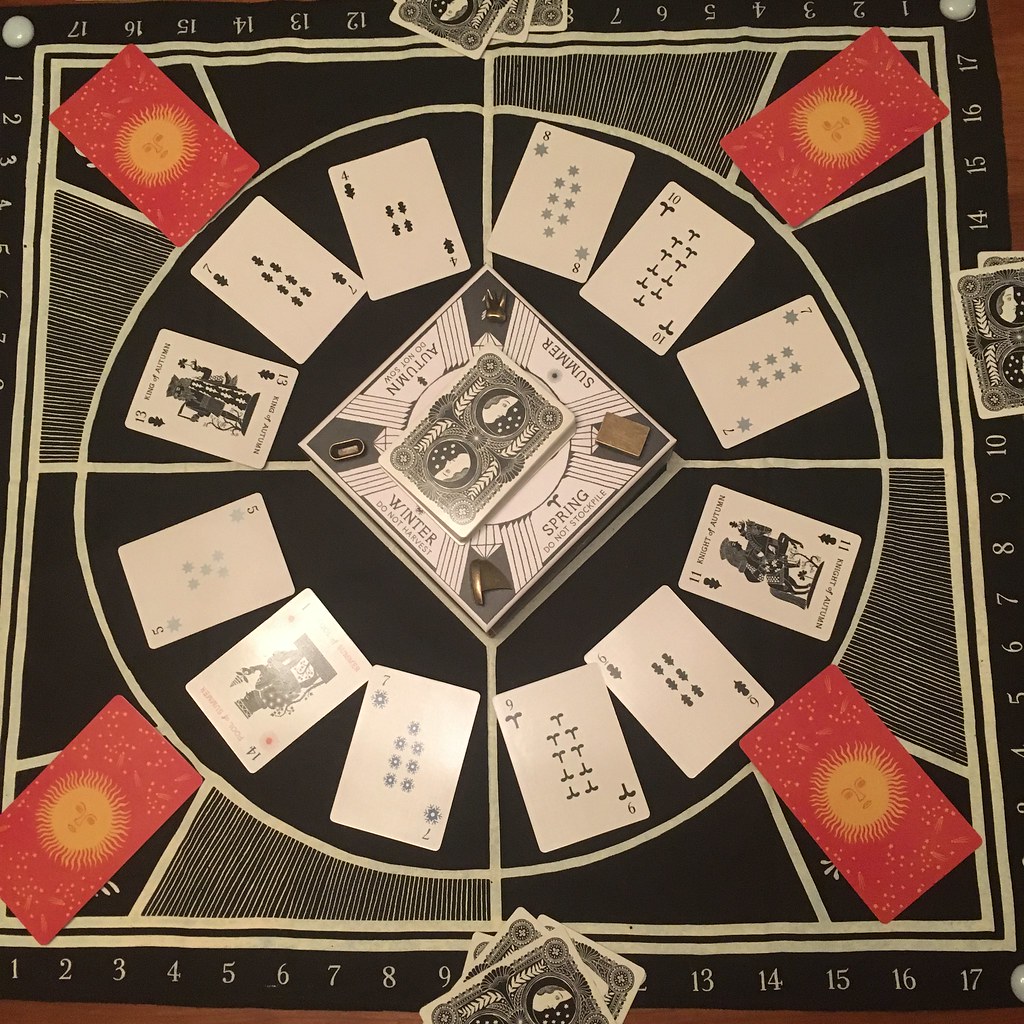In this intricate image, we see an overhead view of a unique game board that appears to be crafted from a large blanket. The background of the scene is predominantly black, providing a stark contrast to the detailed elements within the board. Around the periphery of the board, numbers run along each edge. In the top left corner, the numbers start at 1 and 2 before getting cut off by the edge of the picture. In the bottom left corner, the numbers begin at 1 and continue sequentially up to 17. A stack of cards situated in the middle of the board obscures the number 10.

On the right-hand side of the board, additional numbers ascend towards the top. Centrally positioned is a square that is turned to the side, surrounded by an arrangement of regular playing cards. These cards are positioned within a circular formation. Each card features black and white color schemes, with numbers displayed on them. At each corner of the central square, a card is angled diagonally facing the corner.

These cards are notably red with small white spots and decorated with sun emblems. The sun illustrations feature extensive rays radiating outward in various directions, each centered with a face drawn in the middle. The square in the center of the board is labeled with the four seasons, each side representing: "Spring" at the bottom right, "Winter" at the bottom left, "Autumn" at the upper left, and "Summer" at the upper right.

The board itself is segmented with solid black areas alongside sections adorned with yellow lines. These lines traverse the entire board, rendered in yellow or gray colors. The overall design includes geometric patterns with a square border encompassing a large, central circle, intertwined with straight lines connecting all parts of this elaborate game board.